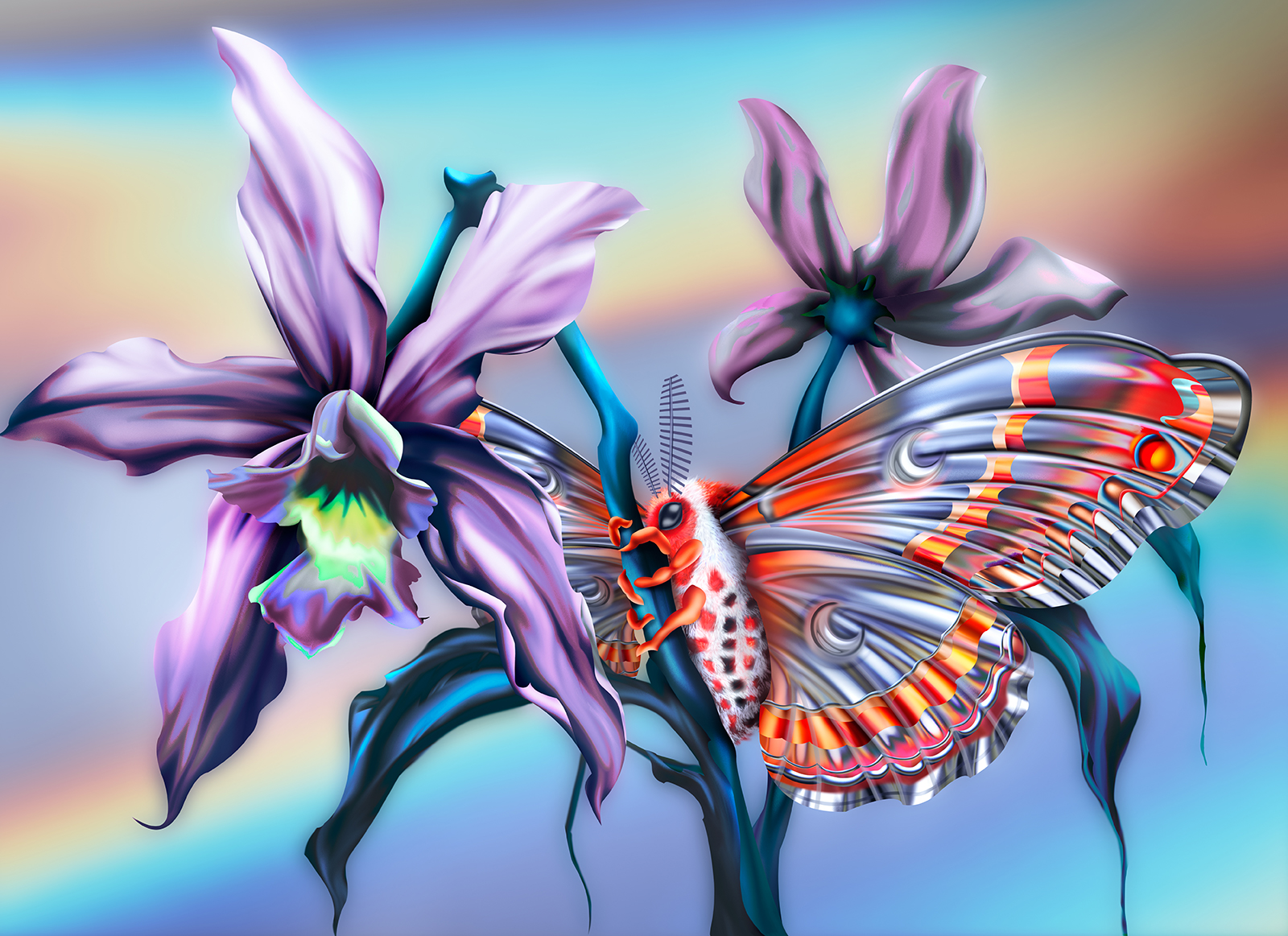This is a captivating and intricate watercolor painting featuring two irises with vibrant blue leaves and branches streaked with purple. The flowers showcase a delicate light purple hue with shades of white, while their inner parts burst in bright yellow and green. A striking butterfly clings to the stem; its legs are a vivid orange, wrapped around the stem, and it has a fuzzy white body adorned with red and black checkered patterns. The butterfly's eyes are surrounded by red, and its wings appear iridescent, with an interplay of pinks, reds, and metallic silver hues that seem almost translucent. The background is a dreamy blur of blue, pink, and purple hues, creating a harmonious and fantasy-like atmosphere. The overall composition suggests a surreal and richly colored scene, filled with a multitude of vibrant shades and intricate details.